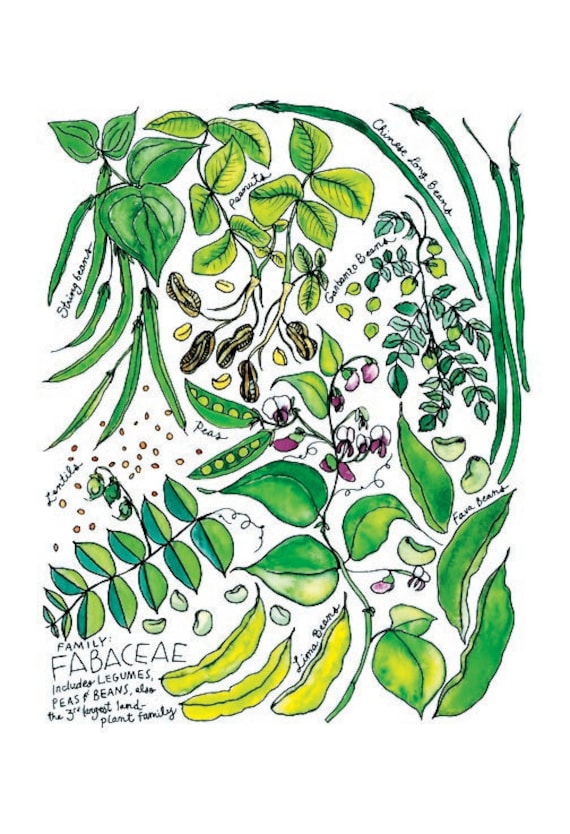This poster is a colorful, cartoonish illustration of various bean plants, showcasing their diverse leaves and features on a white background. The hand-drawn, almost childlike images include string beans, an uprooted peanut plant, garbanzo beans on leafy branches, pods of peas, lima beans, lentils, and fava beans. The leaves depicted range from bright lime green to deep dark green, with a variety of shapes and sizes, adding to the overall diversity. In the lower left corner, the text reads, "Family: Fabaceae, includes legumes, peas, and beans," and mentions that it is the third largest land plant family. The purpose of the poster could be educational, potentially for biology classes or aspiring farmers.